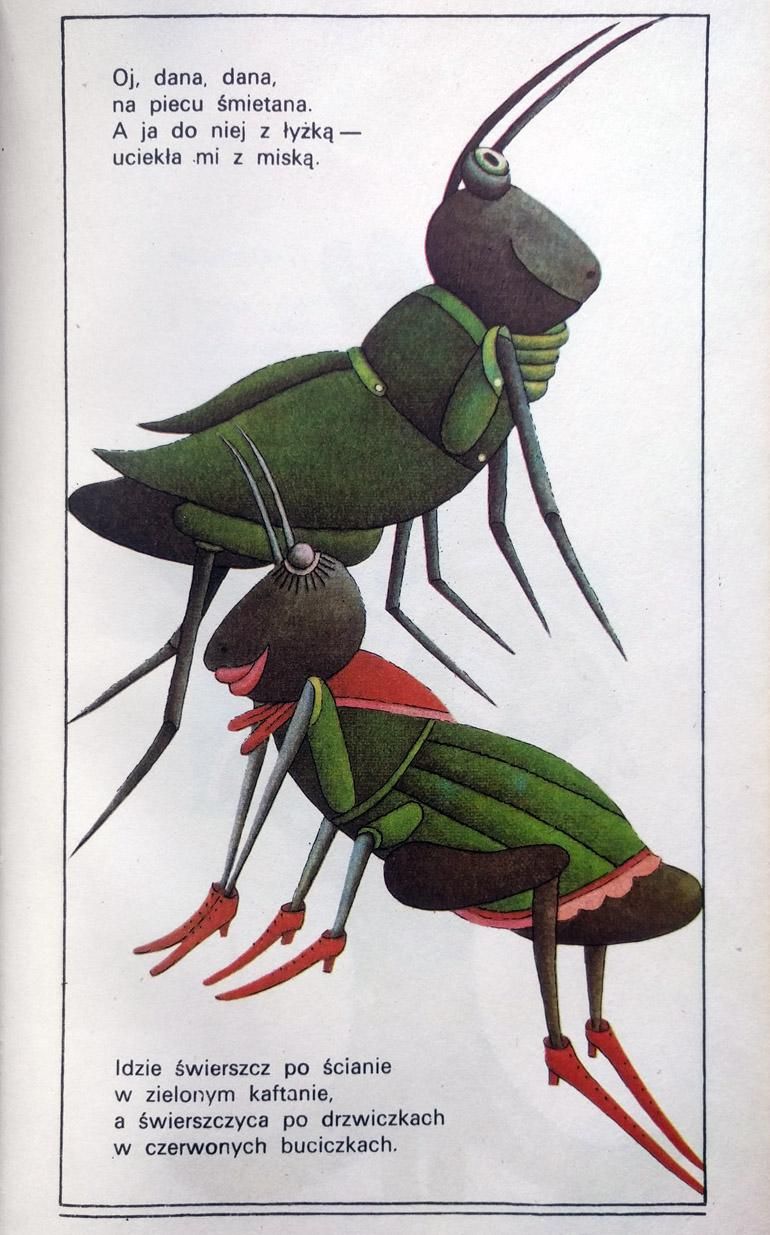This is a detailed illustration likely from an Eastern European children's book or poem, featuring two anthropomorphic insects, possibly crickets or grasshoppers. The scene depicts a male and female insect, distinguishable by their attire and features. The male insect, situated above the female, is facing right and is adorned in green, possibly wearing a vest. His long antennas are black. The female insect, situated below and facing left, is notable for her red lipstick, red high-heeled boots on all six of her feet, and perhaps a dress, along with gray antennas. The illustration employs a gouache-like style and includes text in an unknown Eastern European language—potentially Polish, Russian, or Ukrainian. The text appears in two four-line segments positioned at the top left and bottom left of the page.